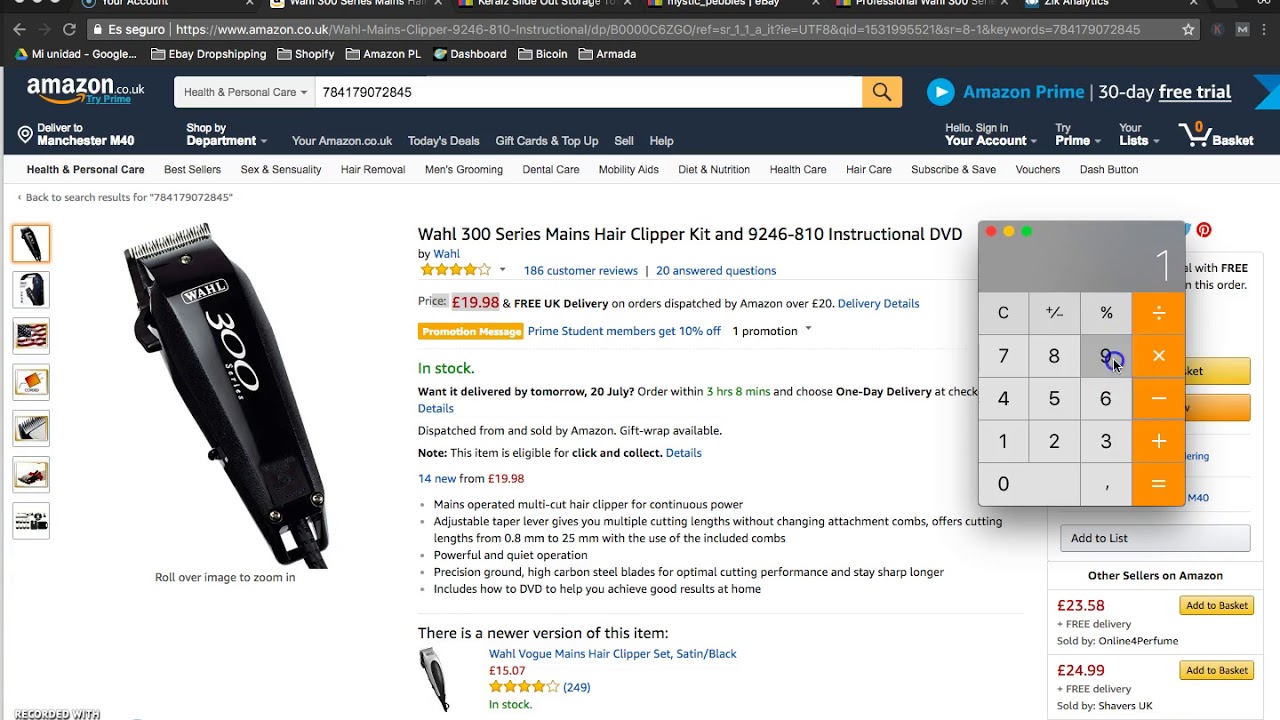Displayed is an image of an Amazon listing on a desktop or laptop screen. The screen shows a calculator overlaying the payment buttons with the number "1" typed into it. At the top of the page, a long white search bar is visible, flanked by menus both above and below it. On the right side, there is a notification for a 30-day free trial of Amazon Prime, along with options for "Your Account," "Try Prime," "Your List," and "Your Basket."

The product listing featured is for a "WAHL 300 Series Man's Hair Clipper Kit and 9246-810 Instructional DVD," though there appears to be a typo referring to "Man's" instead of "Men's." The price, free delivery option, and stock availability status are also displayed. Detailed product information, including specifics about the item, are listed below, next to a main picture of the hair clipper and razor.

On the left side of the information, smaller thumbnail images of the product are arranged vertically, providing alternate views. The overall layout is characteristic of a standard Amazon product page, presenting a comprehensive overview for potential buyers.